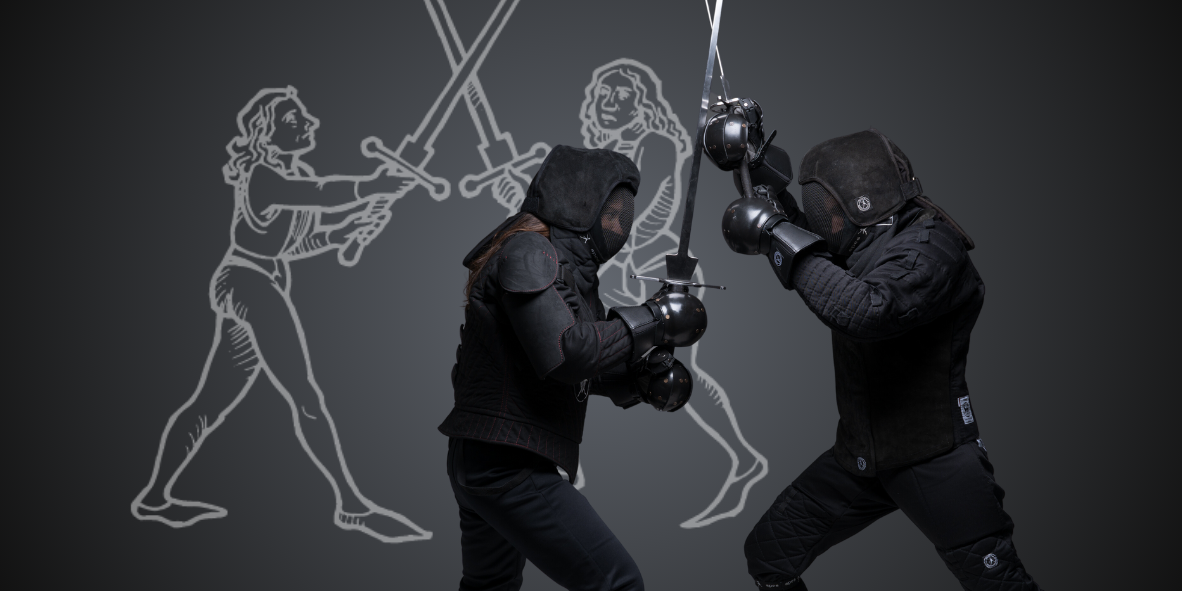This horizontal-rectangular photograph features a dynamic scene of dual sword fighting. In the foreground, two individuals clad in black fencing outfits engage in a duel, each wielding a long silver sword. Both combatants are fully protected with face shields, heavy gloves, and comprehensive black protective gear. One fencer grips the sword with both hands, holding it sideways, while the other prepares for an imminent strike, their swords on the verge of clashing. Both fencers lean into the action with bent knees and legs positioned forward, exuding intensity and focus.

In the background, a dark charcoal gray wall serves as a canvas for a white outline drawing, depicting two figures also in a heated duel. The minimalistic yet powerful illustration shows these figures with long hair and minimal clothing, their massive swords crossed in mid-air. This artistic representation echoes the action in the foreground, creating a visual connection between the real-life fencers and their depicted counterparts, adding depth and context to the energetic scene.